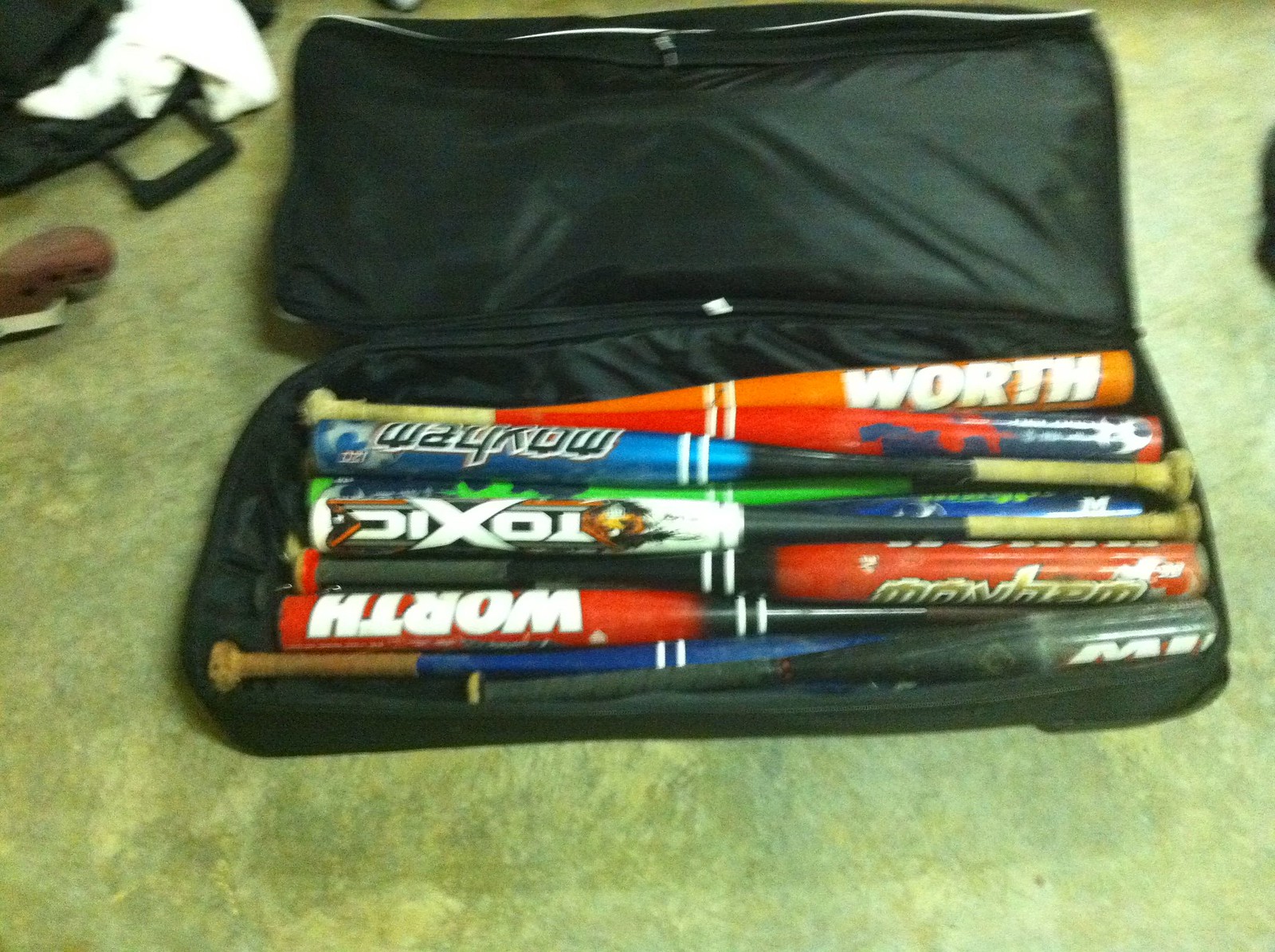This image features a large, soft black sports bag resembling a shallow suitcase, with a padded top that zips open completely. The bag is currently open, revealing an assortment of baseball bats inside. The bag contains roughly 10 to 20 bats, including a notable orange bat with white "Worth" lettering, a black bat with "Toxic" written on it, and a black-and-red bat also labeled "Worth" in the opposite direction. There's also a blue bat with possibly "Mayhem" written on it, and a variety of other bats in colors like green, silver, and multiple shades of red and blue. Most of the bats feature a distinctive double white stripe around the middle where they widen. The bats are placed in alternating directions, filling the bag entirely. The background is a somewhat ambiguous surface—either concrete or an old, dirty gray-green carpet—making it hard to discern the exact material. In the upper left corner of the image, there's another suitcase with a white cloth or shirt draped over its edge, adding to the cluttered scene.